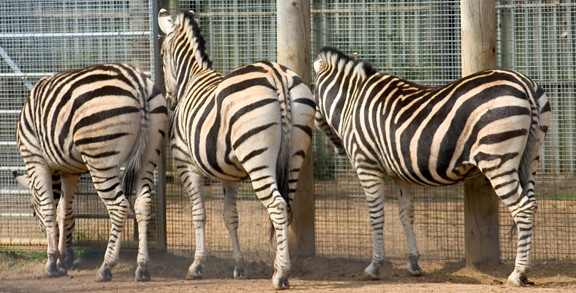In this photograph, three zebras are standing inside an enclosure with their backs to the camera. The enclosure consists of a metal fence with robust wooden poles, and there's a closed metal gate on the left side in the background. The zebra on the left has its head bent down, presumably grazing on some grass growing under the fence. The middle zebra stands upright, facing forward with its head up, while the zebra on the right stands similarly but has its head turned slightly to the right. All three zebras have their tails tucked between their legs and light-colored tails with black tips. None of the zebras are touching each other, and one is slightly more in profile compared to the others, allowing a partial view of its side.